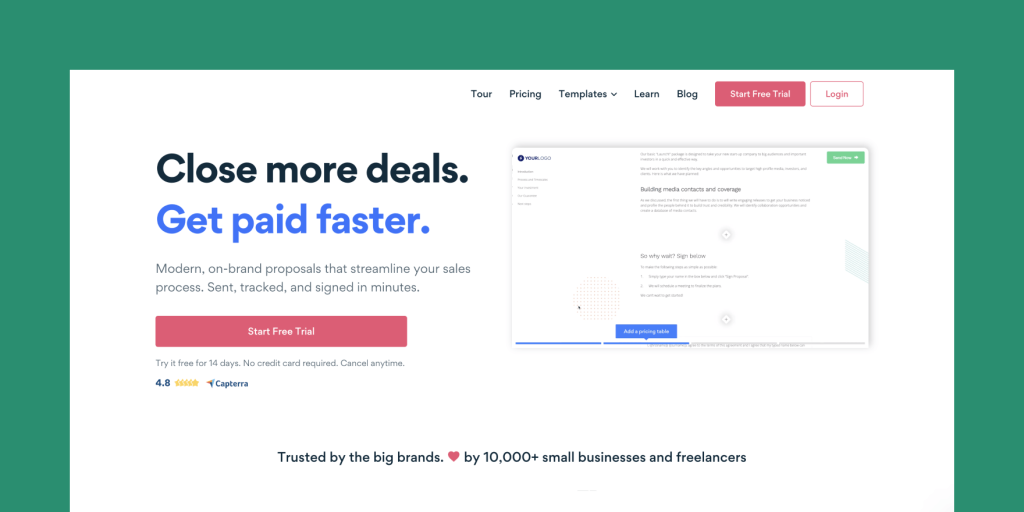Here is a refined and detailed caption for the image described:

---

The screenshot showcases a polished webpage with a dark green background, overlaid by a solid white box in the center. The top-right section of the white box features a navigation bar listing the options: “Tour,” “Pricing,” “Templates” (with a downward arrow indicating a dropdown menu), “Learn,” and “Blog.” Adjacent to these are two buttons: a vibrant pink button labeled “Start Free Trial” in white text, and a second button outlined in pink that reads “Login” in pink text.

On the left side within the white box, the prominent title displays “Close More Deals” in black text and “Get Paid Faster” in blue text. Below the title, a subtitle in smaller font reads: “Modern On-Brand Proposals that Streamline Your Sales Process, Sent, Tracked, and Signed in Minutes.” Positioned underneath, another pink “Start Free Trial” button appears, accompanied by the text: “Try It Free for 14 Days, No Credit Card Required, Cancel Anytime.”

Further down, a rating of 4.8 stars is highlighted alongside the Capterra logo, reflecting user satisfaction. On the right side of the title, there is a visual representation of the "Your Logo" website, which includes sections titled “Building Media Contracts and Coverage” and “Customization.”

Centrally placed at the bottom of the white box, bold black text states, “Trusted by the Big Brands,” followed by a heart emoji, and continues, “by 10,000 plus small businesses and freelancers.”

---